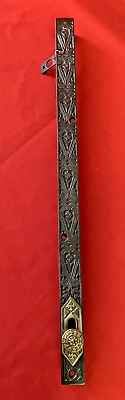The image showcases a detailed product photo by Sony, featuring a long, thin object with ornate carvings, set against a red silk cloth background. The object, which resembles a pencil or perhaps a ruler in shape, is likely made from wood or metal, with intricate design elements. It has a brownish color with gold embellishments and several red jewels adorning its surface. A small red jewel is prominently placed near the bottom, along with a copper or brass fitting integrated into the design. The top part features a clasp or tag with red detail, adding to its ornate appearance. The item includes a slide with a small door-like feature. Although the exact function of this object is unclear, it could be some type of specialized instrument or ceremonial item.